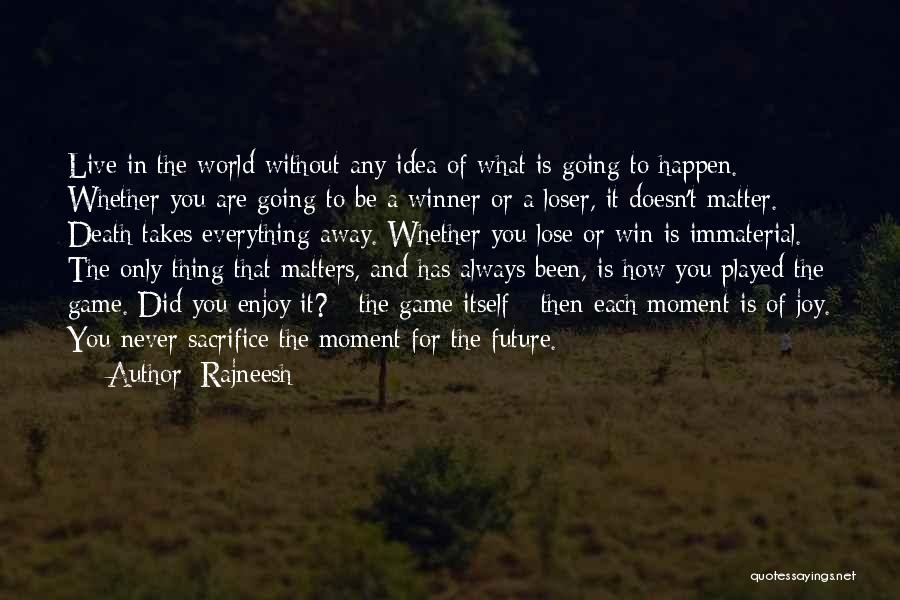The image is a blurry and very dark photograph of a field with beige and green grass, weeds, and small bushes. In the background, under a pitch-black sky, there are larger trees and visible branches on the top left corner. Toward the very far right, there appears to be a person walking to the right, although it is hard to make out clearly. The entire scene has an olive drab green, black, and beige color scheme. Superimposed on this image is a white text quote by Raj Nish, formatted in six lines. The quote reads: "Live in the world without any idea of what is going to happen. Whether you are going to be a winner or a loser, it doesn't matter. Death takes everything away. Whether you lose or win is immaterial. The only thing that matters, and has always been, is how you played the game. Did you enjoy it, the game itself? Then each moment is of joy. You never sacrificed a moment for the future." At the bottom right corner of the image, it says "quote sayings.net" in white text.